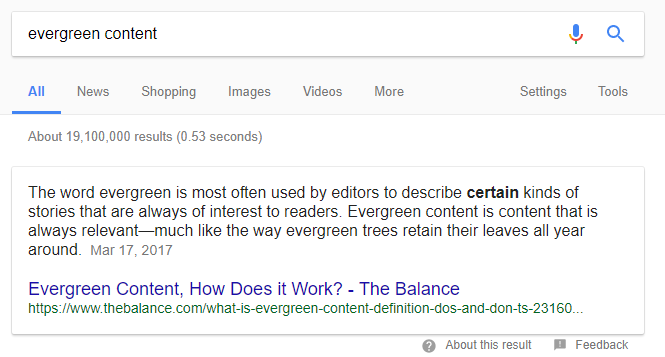This screenshot captures a Google search result page for the query "evergreen content." The rectangular screenshot is small and only shows part of the page, excluding the full content. The background is white, and at the very top, there's a light gray rectangle. Within this rectangle is a white search field with the text "evergreen content" in black font. To the right of the search field are a blue microphone icon and a blue magnifying glass icon.

Below the search field, there are selectable tabs including "All," "News," "Shopping," "Images," "Videos," "More," "Settings," and "Tools." The "All" tab is currently selected. Directly beneath these tabs is a note indicating that approximately 19,100,000 results were found in 0.53 seconds.

Further down, the screenshot displays the outline of a black rectangle enclosing a snippet of information. This snippet includes a black font description: "The word evergreen is most often used by editors to describe certain kinds of stories that are always of interest to readers. Evergreen content is content that is always relevant, much like the way evergreen trees retain their leaves all year round." Below the description, the date "March 17, 2017" is mentioned. At the very bottom part of the screenshot is a search result titled "Evergreen Content: How Does It Work?" from The Balance.